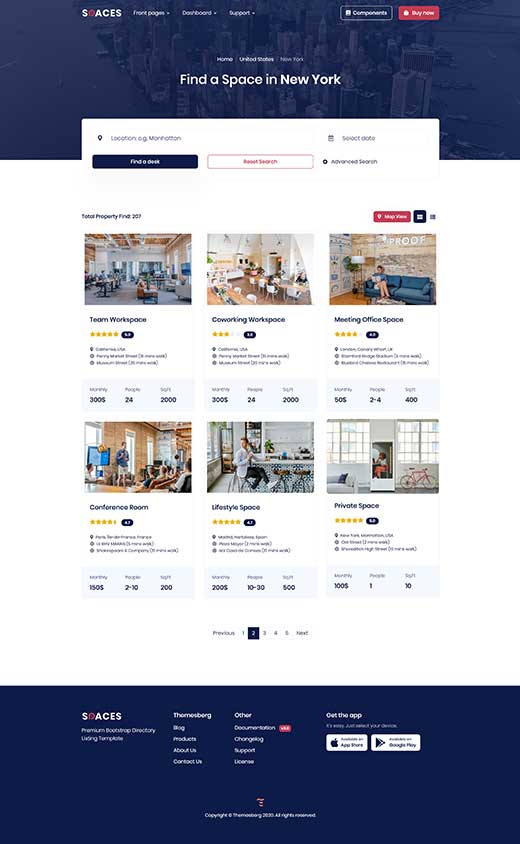The image depicts a full-page view of a website, predominantly featuring a white background without any noticeable borders. At the top, there's a prominent blue banner with the text "Spaces" or possibly "Aces" visible, accompanied by three menu items, each with drop-down arrows indicating further selections.

On the right-hand side, two rectangular boxes are visible, each containing distinct content. The first box is red and includes a "Buy Now" call to action. Below this, centered on the page, is the phrase "Find a space in New York," superimposed on a vague cityscape backdrop resembling Manhattan. Within a white area of the page, there are two buttons: one blue rectangular button and one smaller white button, accompanied by a small icon.

Further down, a section showcases six media images, each paired with a rating. The categories and their corresponding images are:
1. "Team Workshop" - Image depicts a collaborative workspace.
2. "Co-Working Space" - Specific details not provided but implies a shared office environment.
3. "Meeting Office Space" - Shows a woman sitting cross-legged on a blue couch.
4. "Conference Room" - Features people in a spacious room with high ceilings and long windows.
5. "Lifestyle Space" - Specific details not provided, likely depicts a versatile working environment.
6. "Private Space" - Specific details not provided, suggests a secluded workspace.

Each of these images is tied to a descriptive heading, offering a visual and textual overview of the spaces available on the site.